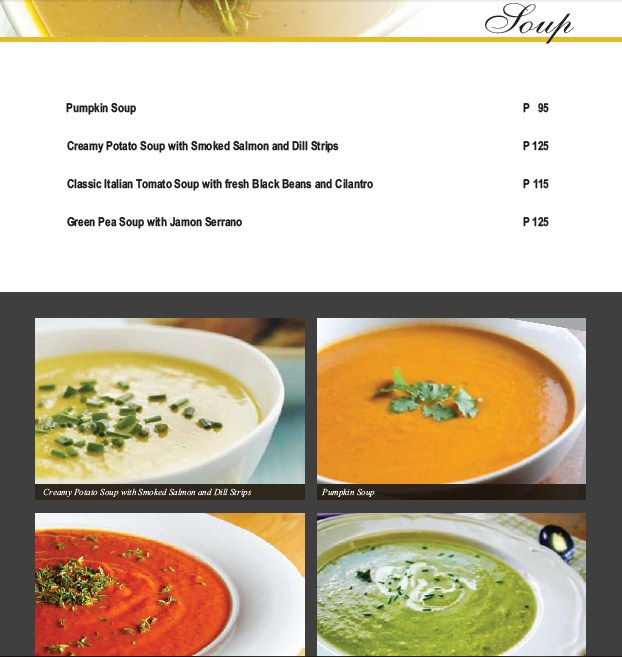This image features a detailed menu page dedicated to soups, masterfully designed with a combination of text and visuals. In the upper right corner, the word "Soup" is elegantly written in a flowing cursive font, accompanied by a partial image of a yellow-hued soup garnished with green herbs. Below this heading, a soft yellow line demarcates the start of the menu items listed with their corresponding prices: 

- Pumpkin Soup (P95)
- Creamy Potato Soup with Smoked Salmon and Dill Strips (P125)
- Classic Italian Tomato Soup with Fresh Black Beans and Cilantro (P115)
- Green Pea Soup with Jamon Serrano (P125)

Under the list, there are four vivid pictures of the soups. From a top-down view and positioned against varied backgrounds—ranging from wooden to blue tables—these soups are displayed in white bowls, exuding a homey yet elegant vibe. The upper-left image features the creamy potato soup adorned with dill strips. To its right, the pumpkin soup appears with a central parsley garnish. The bottom-left image shows the classic Italian tomato soup with a possible garnish of basil or oregano. Finally, the bottom-right image illustrates the green pea soup, sprinkled with either parsley or chives, and elegantly presented on a slightly more ornate white bowl with an accompanying spoon and placemat. The visual arrangement is reminiscent of a well-crafted window panel, immersing the viewer in the diverse and appetizing world of soups.